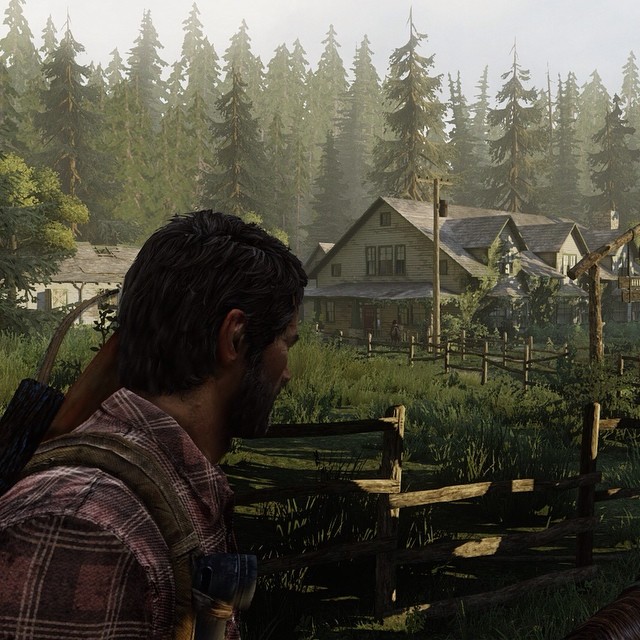The image captures a moment from a video game, depicting a serene yet eerie wooded environment. In the background, a foggy sky casts a grey hue over low-detailed, vividly green pine trees, creating a misty and atmospheric setting. The foreground features the back and shoulder of a male character, viewed from over his right shoulder. He is dressed in a red and black flannel shirt and has brown, short hair with a beard, identifying him as a white male. Slung over his right shoulder is what appears to be a bow and quiver, suggesting he is prepared for survival or hunting.

The character's gaze is fixed on an old, weather-beaten wooden house situated on the right side of the image. The house appears to be in a state of decay, with visible signs of rotting wood. A wooden fence starts from the left side of the image, curving along a pathway towards the right, and then winding back towards the house at the center. The overall composition and elements contribute to a feeling of anticipation and exploration within the game.